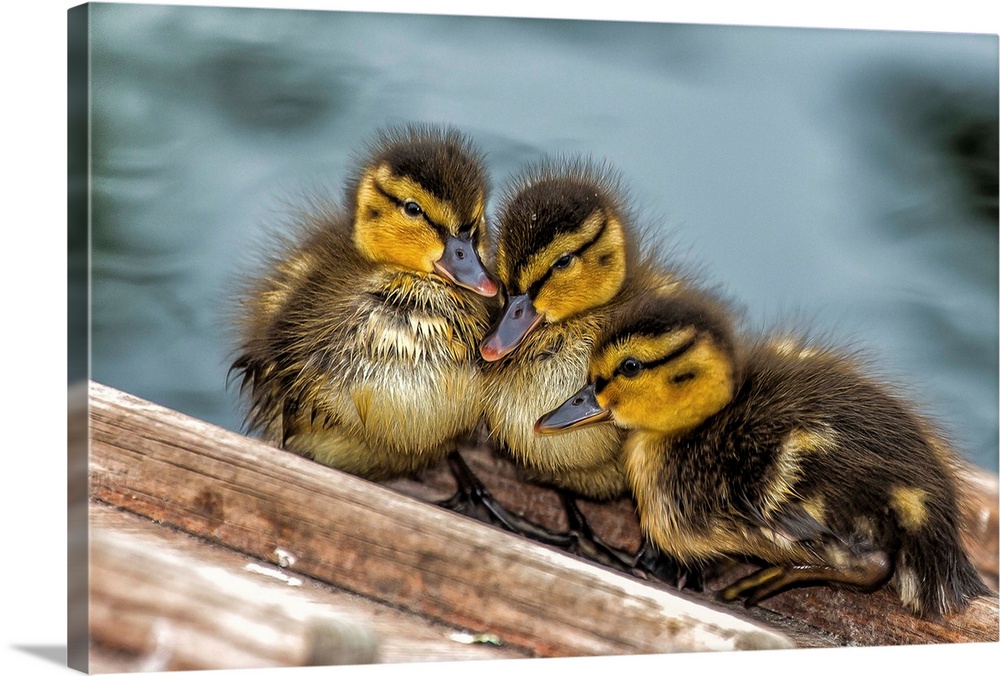In this image, three young ducklings, possibly mallards, are perched together on what appears to be a wooden bench or deck. The ducklings exhibit a mix of brown, yellow, and black hues, with distinctive yellow heads and black markings around their eyes. Their beaks feature a gradient of colors, primarily black with hints of gray and orange, while their feet are black. The feathers on their bodies display a spiked pattern of brown and yellow, with a notable black streak running through their eyes to the back of their heads, giving them a mohawk-like appearance. They seem to be waiting for food, with their beaks pointed towards the left side of the image. The wooden surface they are sitting on is brown, and the background behind them is a blurred mix of dark shades, including gray, brown, and black, creating a somber mood. No text is visible in the picture, and the primary colors observed are yellow, black, and various shades of brown and gray.